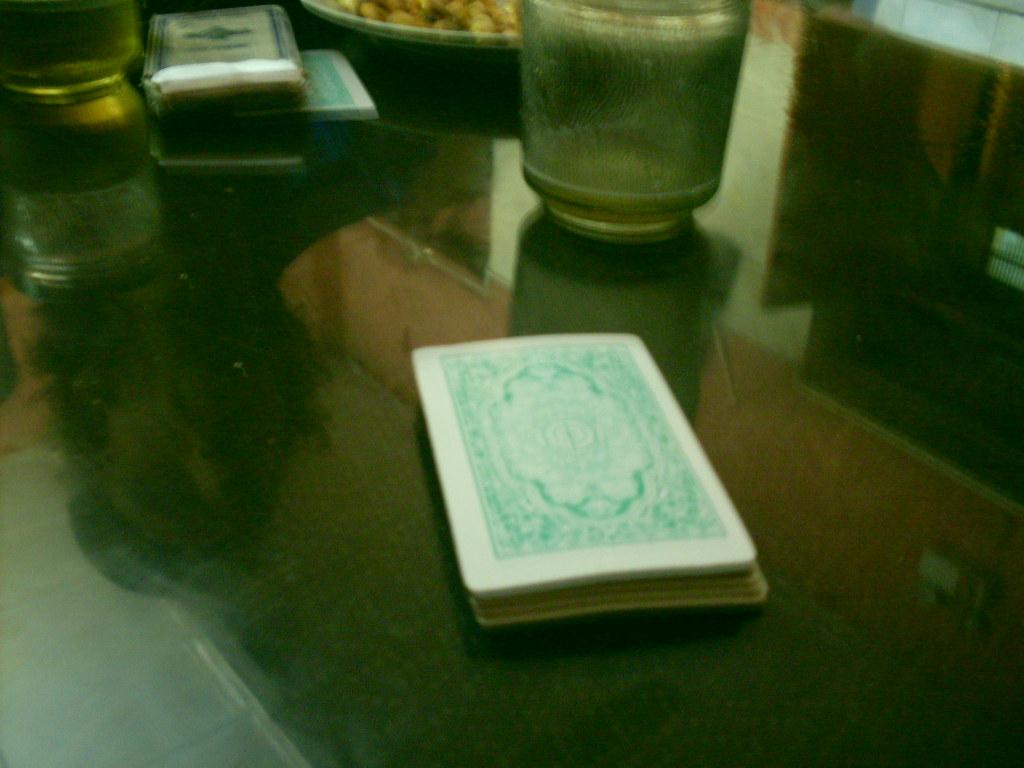In this low-quality, blurry photograph, the entire background is dominated by a shiny green surface, possibly a table at a restaurant. Reflected on this glossy surface is a vague image of the photographer, a Caucasian individual with shaggy hair, intently looking down. At the center of the table lies a deck of cards, stacked neatly with their backs visible. The card back design is intricate, resembling a Persian carpet in red. To the right, a frosted glass cup sits, its contents indiscernible due to the poor quality of the image. On the opposite side, in the upper left corner of the table, another deck of cards is visible, accompanied by a glass that appears to contain beer.